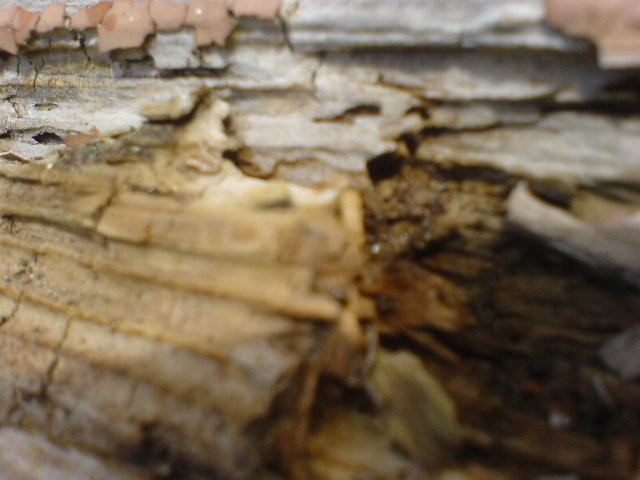The image is a detailed close-up of a weathered piece of bark, possibly from an old log, set in an outdoor environment. The bark is broken and chipped, revealing jagged, darkened, and aged wood beneath. Different shades of brown dominate the wood, with the darkest areas clustered in the lower right, contrasting against lighter browns towards the right edge. The bark’s surface is irregular and marked with numerous chips, suggesting it has endured extensive wear. In the background, at the top left, remnants of an orangey-brown tiled structure, possibly a roof or fence, are visible. Behind the tiles, aged and patchy white concrete adds to the rustic outdoor ambiance.